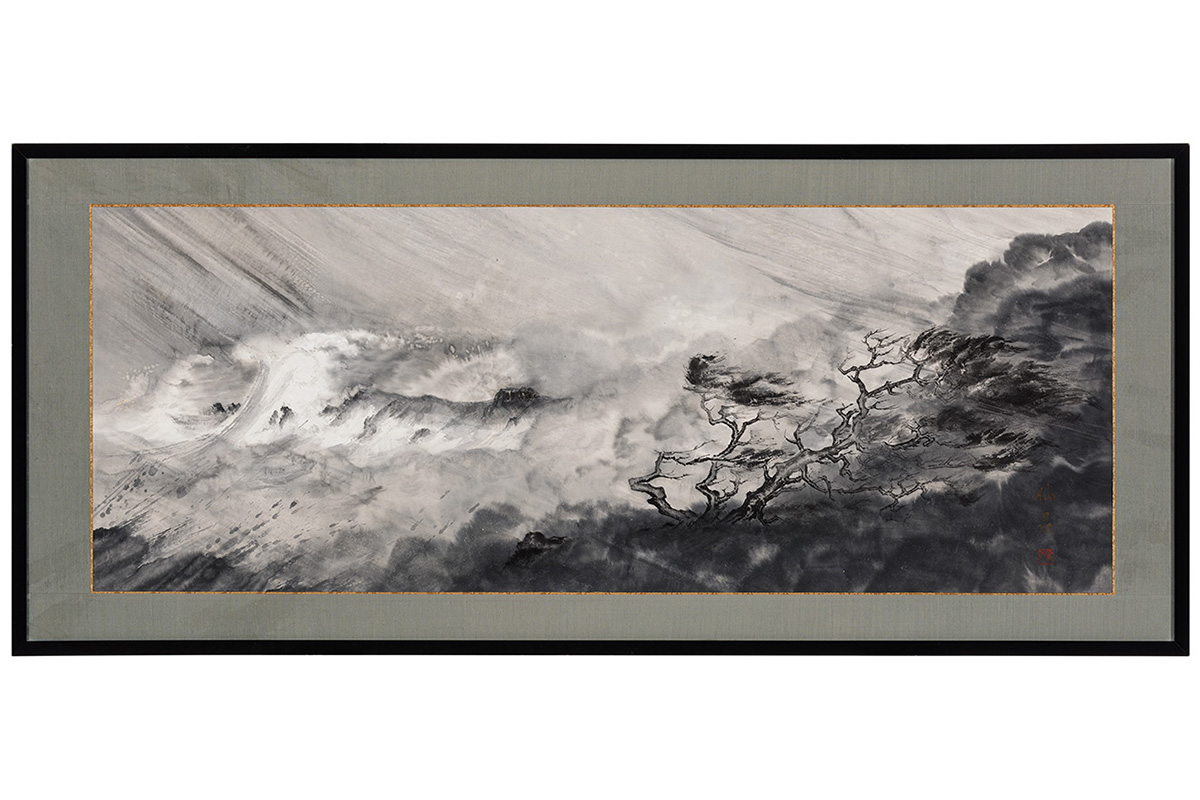A striking horizontal illustration framed in black, with a gray fabric-like border and adorned with a gold trim, showcases a dramatic storm scene. On the right side of the image, gnarled trees bend under the force of a powerful wind, leaves swept to the right. The dark surface beneath the trees suggests a grass-covered landscape. To the left, tumultuous waters feature varying shades of gray, black, and white, with waves crashing amidst the chaos. The sky above is streaked with dark lines, all seemingly driven towards the right, enhancing the sense of ferocity. Additionally, scattered stones appear in the bottom left corner, completing this monochromatic depiction of nature's fury.